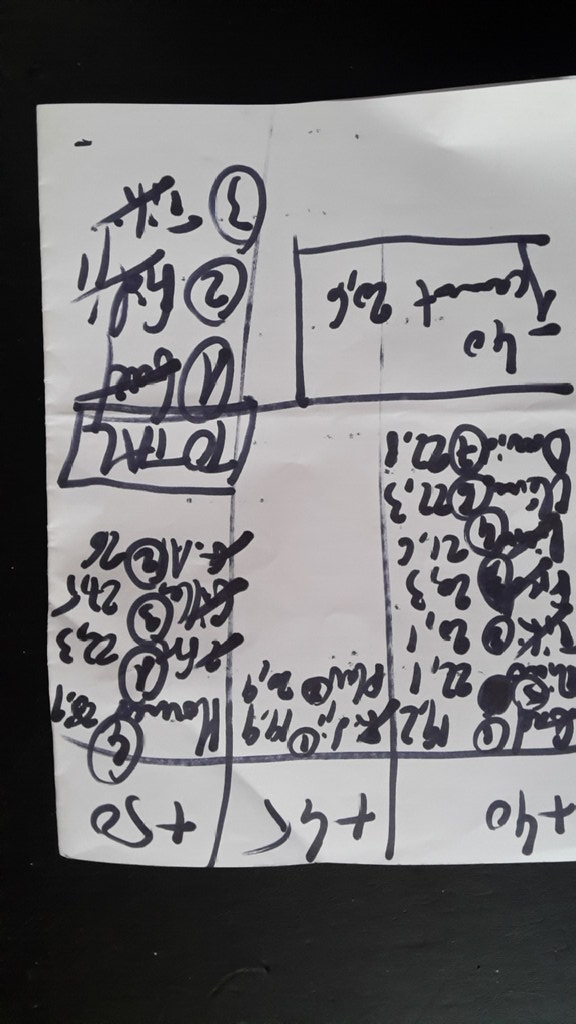The image depicts a creased and crinkled white piece of scratch paper, which appears to have been written on using a thick black permanent marker. The text on the paper, though somewhat disorganized and with some characters upside down, includes both numbers and words. The numerals "+40," "+45," and "+50," along with the word "total" in English, stand out amidst the various handwritten columns. These columns, though freehand and not symmetrically drawn, give the impression of a makeshift table used for some form of tracking or calculation, possibly reminiscent of a tally sheet from a restaurant host's stand or a casual way to keep track of prices or counts.

Some numbers on the paper have been circled, while others are crossed out, indicating that the document has seen multiple updates over time. Certain parts of the text are legible, while others are either obscured, illegible, or possibly written in a language other than English. The paper seems to have been folded and unfolded, as evidenced by the visible creases. The entire document is photographed against a stark black background, further highlighting the makeshift nature of this rough, utilitarian record-keeping tool.